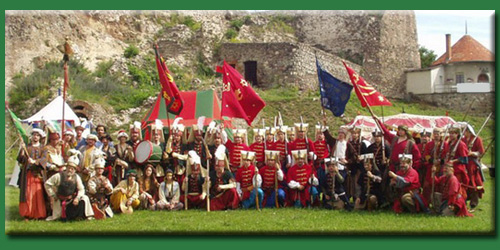The photograph captures a lively medieval reenactment event set against the backdrop of a stone-built medieval structure with a small doorway and a more modern building with a brick roof, both nestled next to a mountainside. Groups of reenactors, vividly dressed in various historical garb, are positioned in the foreground on a grassy area. They are arranged in rows for the photograph, with some kneeling and others standing, many holding flags of distinct colors: a red and yellow flag, a dark blue flag, a red flag held by a group in gold jackets and blue pants, another red flag held by a group in red and green attire, and a group in white with pointy hats holding a flagstick without a visible flag. The participants are equipped with period-appropriate weapons like swords and guns, enhancing the historical ambiance of the scene.